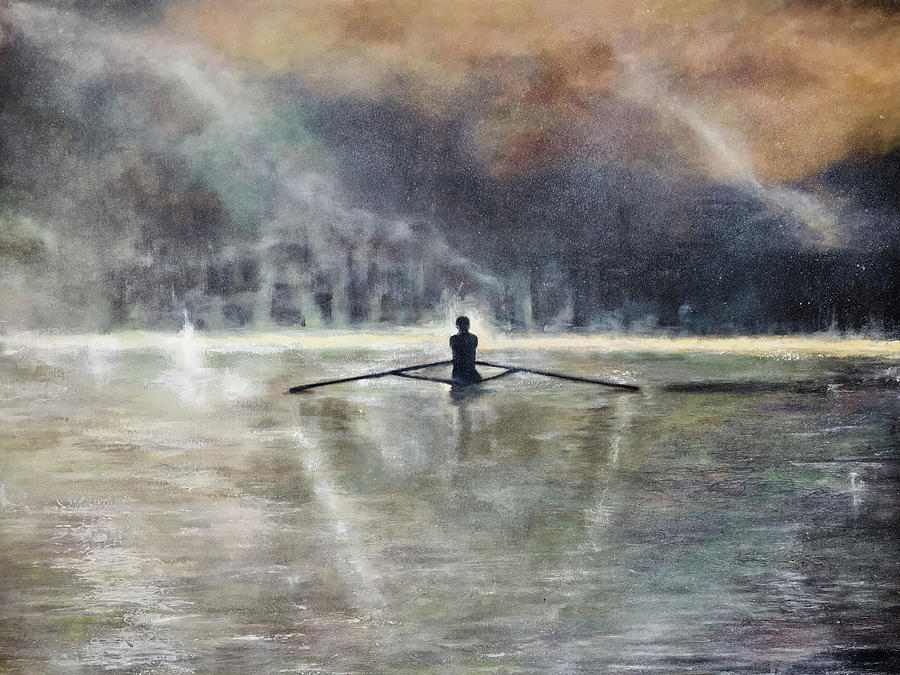The image is an artistic, stylized painting portraying a black silhouette of a person rowing a boat on an abstract waterway. The person, small in comparison to the expansive scene, appears positioned near the horizon, almost in the distance. The composition features striking contrasts, with the ocean painted in sandy beige, green, and dark blue hues, resembling a metallic sheen in grays and blues. The sky overhead is dark and moody, blending night-time grays and stormy browns, with splashes of color reminiscent of an aurora. The central focus is the rower, framed within the middle of a diamond shape formed by diagonal lines, creating a sense of movement and depth. The image is imbued with muted yellows, greens, purples, and oranges, giving it an overall melancholic yet compelling atmosphere.